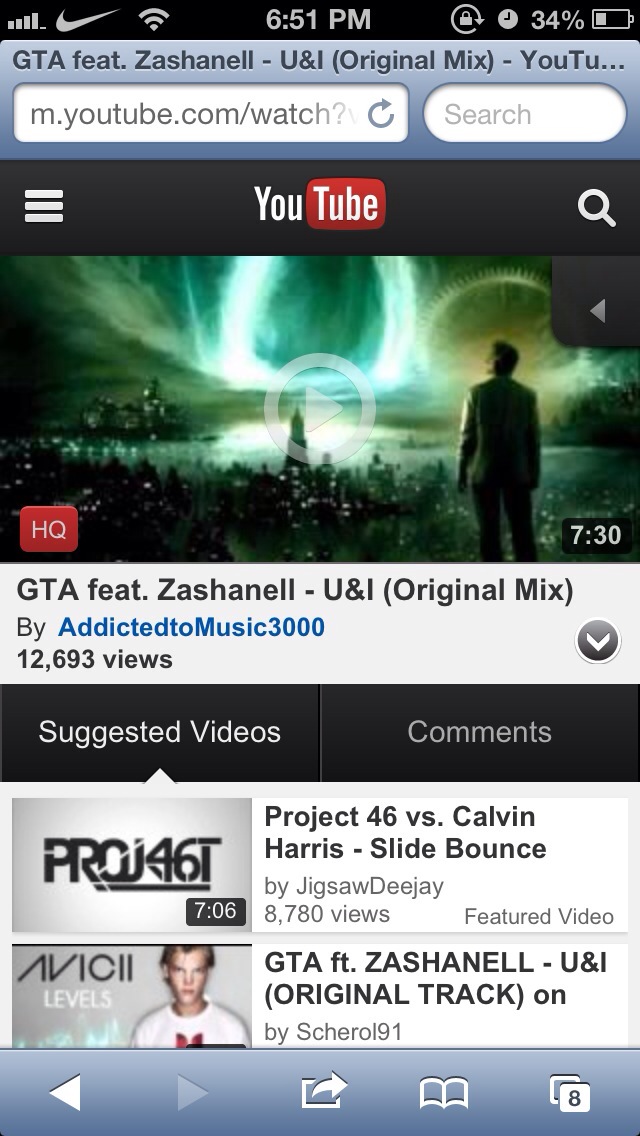The image is a screenshot taken from a mobile phone displaying a YouTube video page in Safari. The main video thumbnail features an artistic representation of a man gazing at a bright, swirling light in the sky above a cityscape. This video, titled "GTA Featuring Zachanel U&I Original Mix," is uploaded by AddictionedMusic3000 and has garnered 12,693 views. The video's duration is 7 minutes and 30 seconds, and it is marked with an "HQ" in the bottom left corner, suggesting high quality. The YouTube interface is predominantly grey and red with hints of blue at the top and bottom of the screen. At the top of the page, the time is shown as 6:51 p.m., alongside Wi-Fi and signal bars, and a battery icon indicating 34% charge. Also visible are the Nike symbol and a search bar. Below the main video, two suggested videos are listed: "Project 46 vs Calvin Harris - Slide Bounce" and "GTA Featuring Zachanel - UI Original Track On." The screenshot seems to depict an older version of the YouTube mobile site.